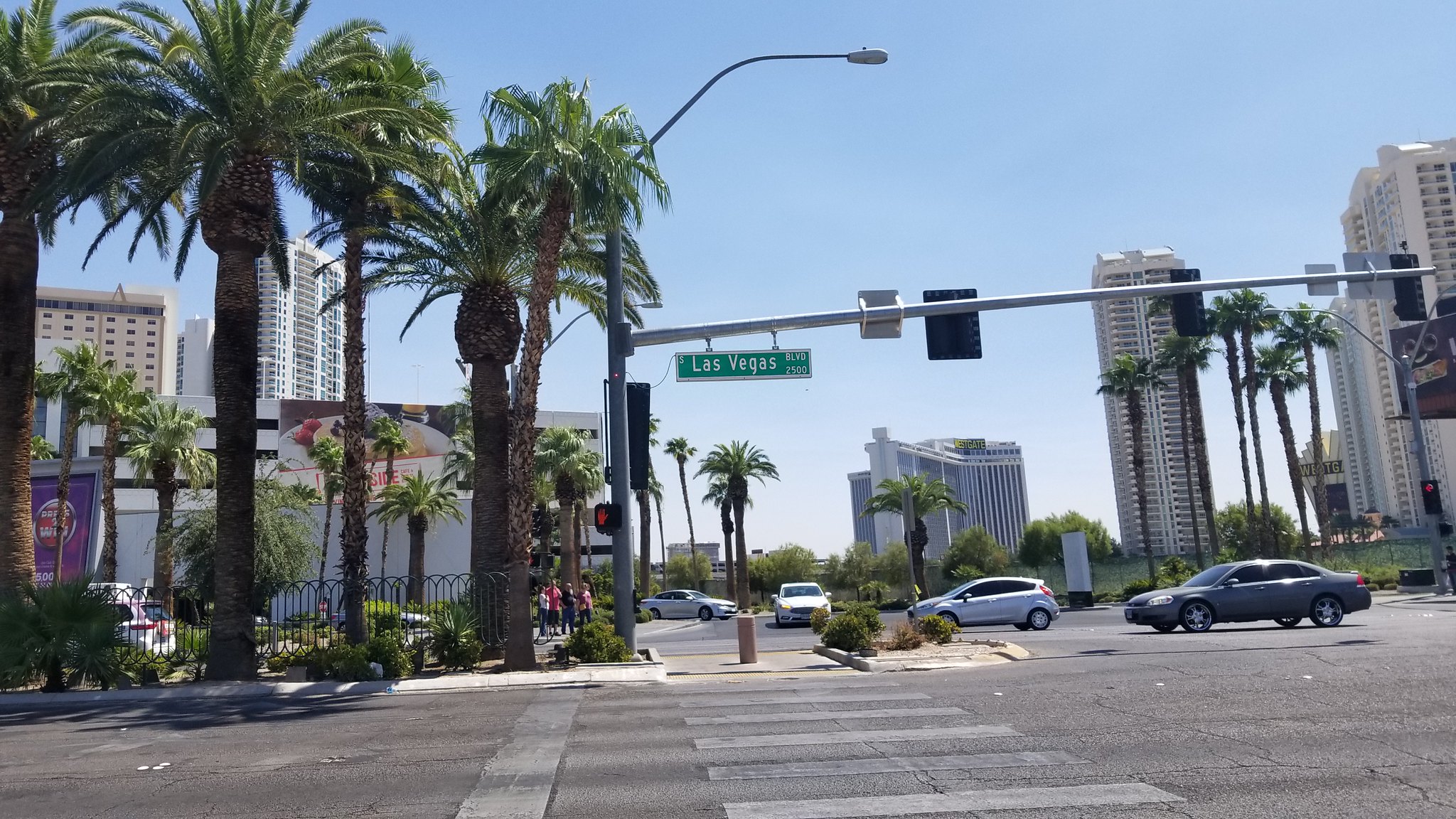This daytime photograph captures a bustling street scene in what appears to be Las Vegas, characterized by its distinctive landmarks and vibrant atmosphere. A rectangular green street sign with white letters prominently displays the name "Las Vegas." Situated nearby is a functioning stoplight directing the flow of traffic and a white-striped crosswalk facilitating pedestrian movement. The backdrop features several tall high-rise buildings in a mix of white and tan hues, reflecting the city's diverse architectural styles. Approximately 20 palm trees line the street, adding a touch of greenery to the urban landscape. Various people are casually standing on the sidewalk, contributing to the lively street ambiance. Multiple cars are present, including a silver van and two white cars parked in close proximity to each other, accentuating the area's high traffic density.